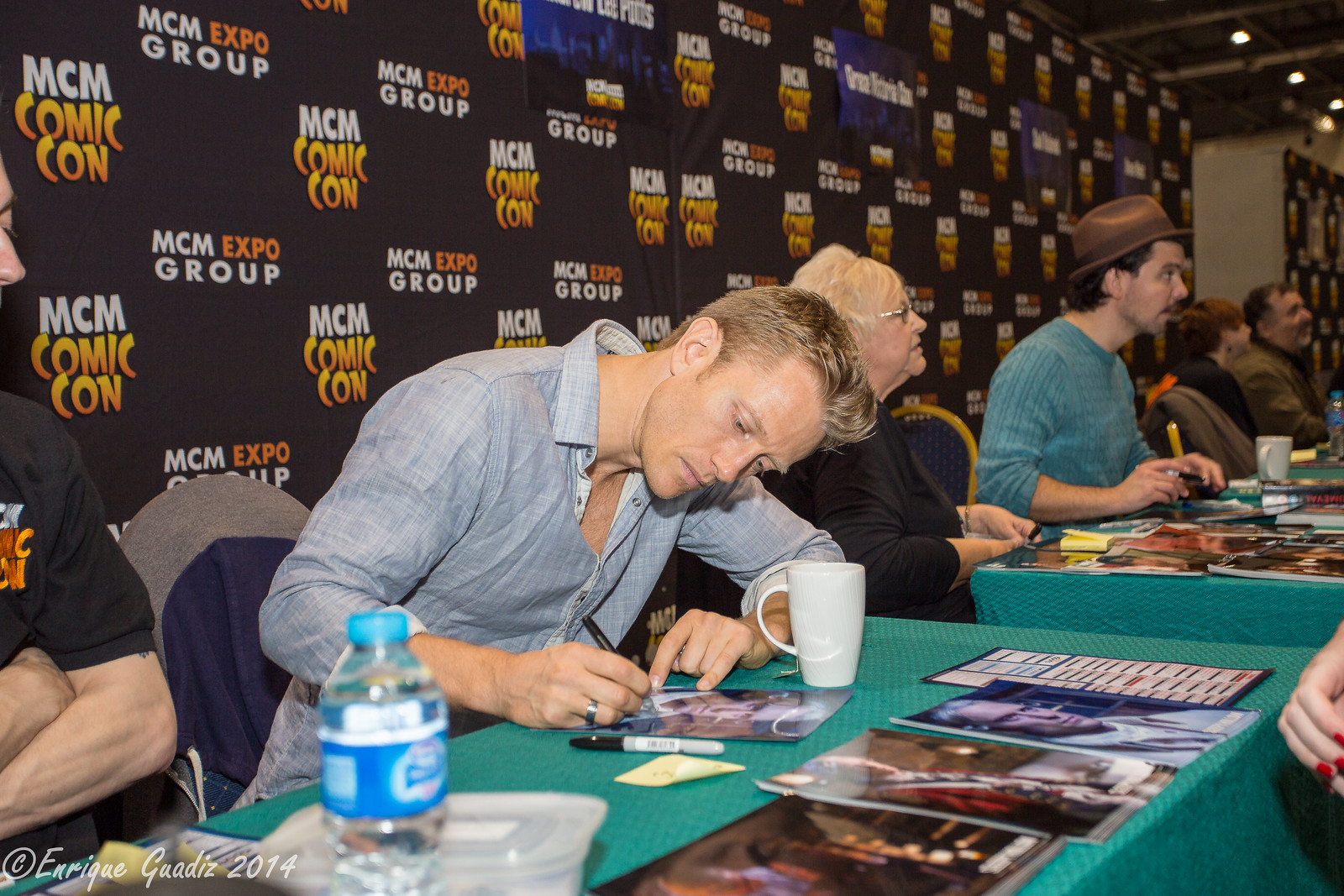The image depicts a lively scene at the MCM Comic-Con, clearly identifiable by the prominent backdrop featuring repeated text: "MCM Expo Group" in white and orange, and "MCM Comic Con" in yellow. The setting is a bustling convention hall filled with tables and a diverse crowd of attendees. At the forefront, a man in a linen button-up shirt is captured in the act of autographing a picture, likely a headshot, with a white cup beside him. To his immediate right sits a woman next to a man donning a brown hat and a greenish sweater. Further along the table, additional individuals including an elderly woman, a redheaded woman, and a bearded man can be seen. Particularly notable is the person sitting to the far left, distinguishable by a black shirt bearing the MCM Comic Con logo and folded arms. The gathered panel of six individuals, likely comprising stars or comic creators, are engaging with the crowd from behind their table filled with signed photographs.